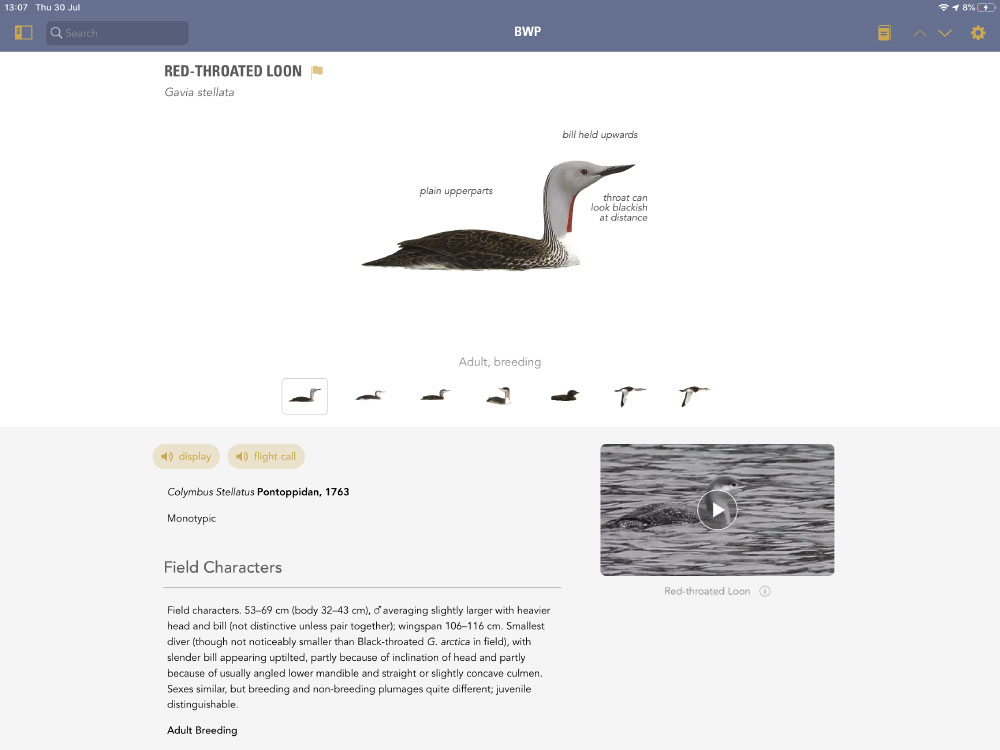Detailed Description of the Website Featuring the Red-Throated Loon:

The screen captures an informative webpage from a site identified by "BWP" at the top. The interface includes a search bar situated on the left-hand side, with a backdrop colored in soft blue hues, setting a calm and serene vibe. 

Prominently displayed, the main section of the page is dedicated to the Red-Throated Loon, scientifically known as *Gavia stellata*. An image of this elegant bird dominates the center stage, presenting the loon serenely nestled in the water. Although the water is not visible, the loon's body is fully showcased. Specific parts of the bird's anatomy are carefully labeled; its bill is held upwards, pointing towards the sky. The bird features a striking white neck and face contrasted by a dark gray plumage covering its back. Notably, a thin strip of red adorns its throat, although an accompanying note mentions that this red marking may appear blackish when viewed from a distance.

Further down the page, additional images capture different views of the Red-Throated Loon, including some displaying the bird in mid-flight. Scrolling down reveals more comprehensive information about the species, such as detailed descriptions, characteristics, behaviors, and other pertinent data, enriching the viewer's understanding of this fascinating bird.